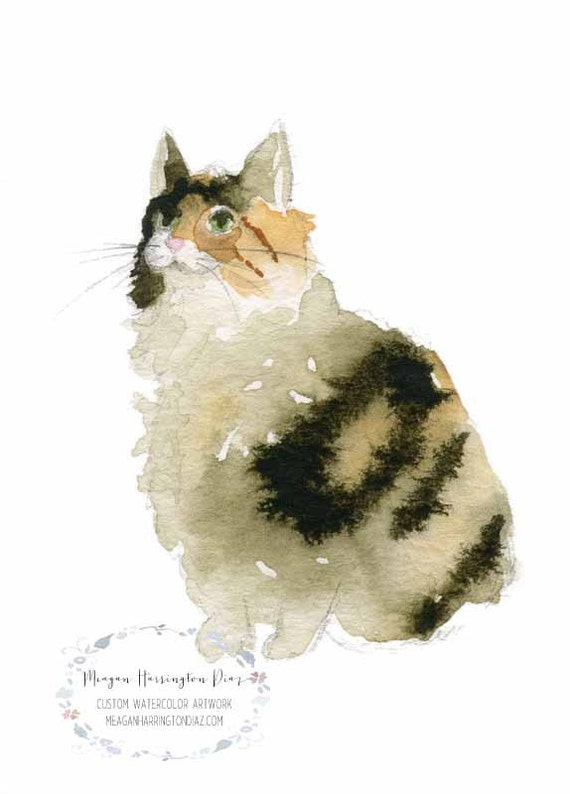The image displays a detailed watercolor painting of a long-haired calico cat in portrait orientation. The cat, seated on its hind legs with its front paws gracefully positioned in front of its chest, is rendered in an array of colors including muddy brown, darkish green, regular green, pink, and light brownish orange. Its head features reddish-brown hair around its cheeks and nose, while its ears are a light gray color and pointed upwards. Remarkably, the cat's eyes are a striking green, with a white nose and black nostrils. The cat's fur exhibits a greenish hue with black spots, complemented by a cream-colored back adorned with black stripes. The painting is set against a white background, and the cat gazes upward and to the left side of the image.

In the bottom left corner, there is an elliptical logo framed by a floral design. Within this border, the artist's name, "Megan Harrison Diaz," is inscribed in black script. Below the name, in smaller gray text, the phrase "Custom Watercolor Artwork" along with the website "MeganHarrisonDiaz.com" is clearly visible. The artwork is a testament to the intricate and vibrant style of watercolor painting.